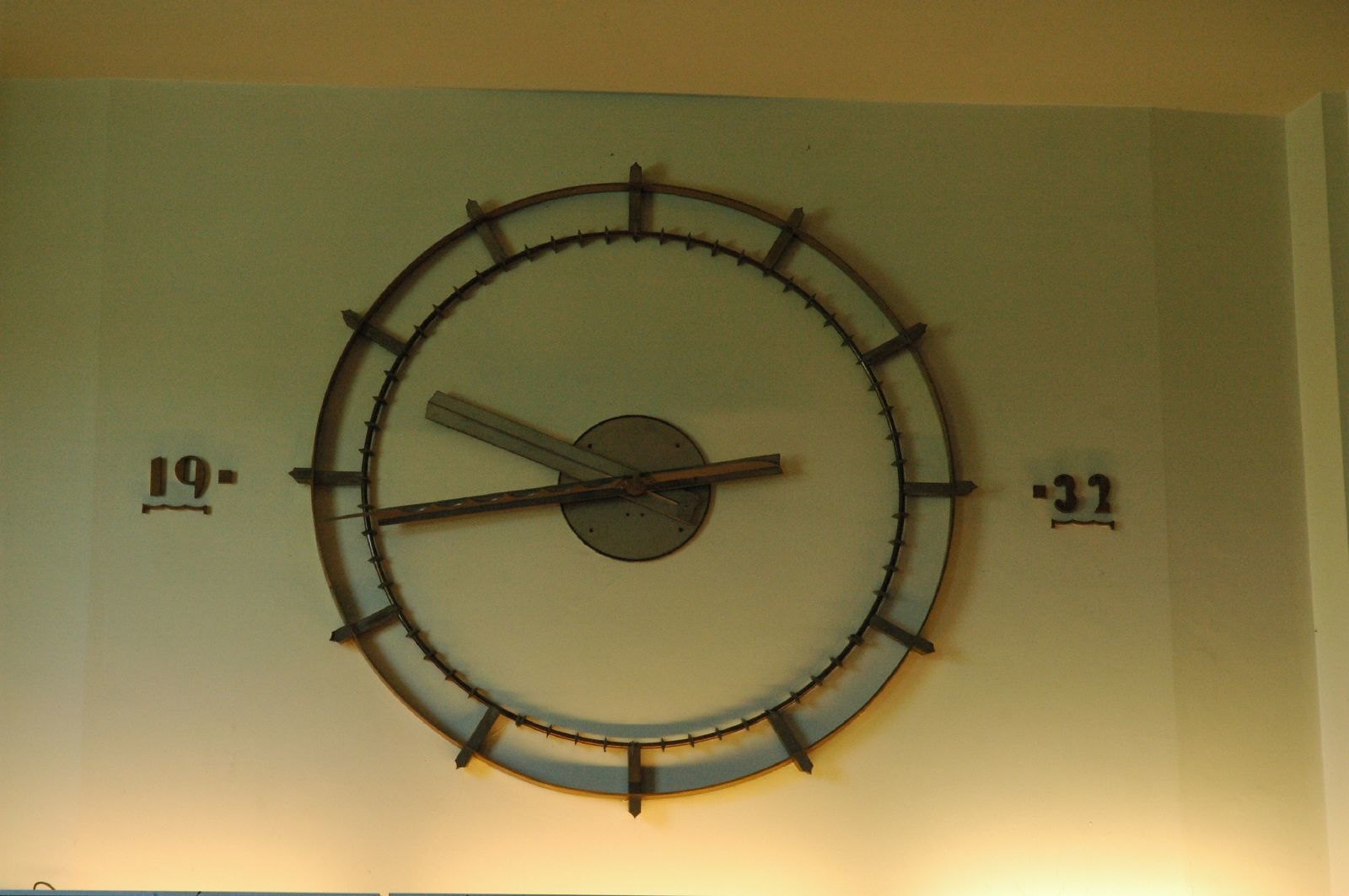The image displays a large wall clock mounted on a green wall, with a yellow ceiling visible above. The clock itself is an art installation comprising two concentric metal circles. The inner circle holds two hands: one appears to be a metal bar, and the other looks like a wooden stick. These hands indicate the time as roughly 9:44. The clock lacks traditional numbers or numerals, instead featuring long dashes to mark the hours. Uniquely, where you would expect the 3 o'clock and 9 o'clock positions, there are wooden numerals "32" and "19" respectively, both underlined with squiggly marks. These digits create a curious contrast and add an intriguing element to the minimalist design. The clock is situated on what appears to be a panel rather than directly on the wall itself.